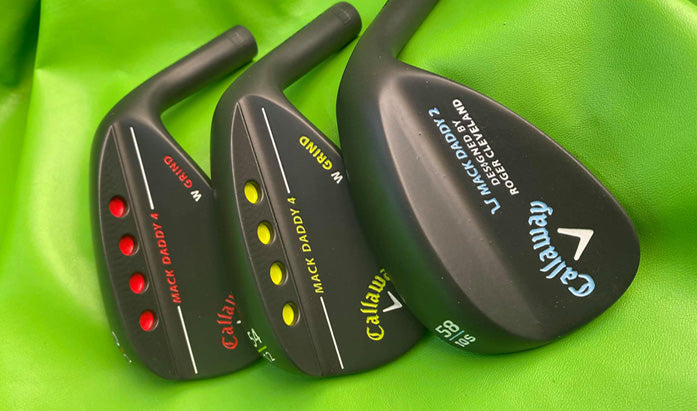This color photograph features three Callaway golf club heads arranged in a staggered layout on a bright neon green cloth, possibly silk or leather, that is slightly folded. The bottom-most club head on the left has red detailing, including the text "Mac Daddy," "Callaway," and "W Grind," accompanied by four red circular cutouts. The middle club head has similar features but replaces the red accents with neon green colors, and includes the text "Mac Daddy 4." The top club head, which differs slightly, has light blue detailing, lacks the circular cutouts, and includes the text "Callaway Mac Daddy II," "58," and "105," along with a note that it was designed by Roger Cleveland.